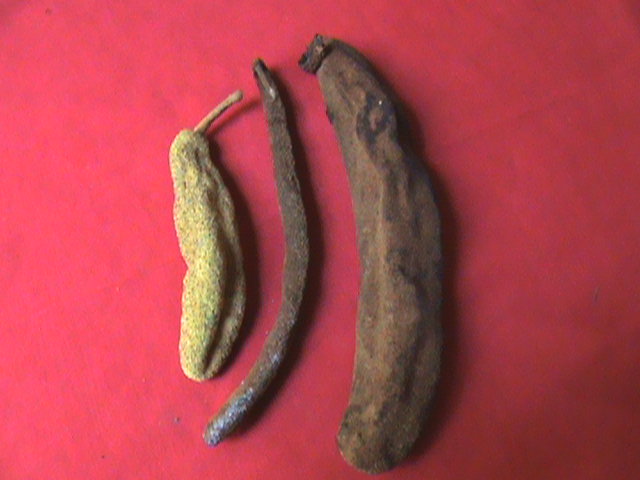The image depicts three very dry and shriveled items that resemble old vegetables or fruits, placed on what appears to be a red background or red construction paper. On the left, there is a slender, yellow, shriveled item, likely resembling a dried pepper. In the middle, there's a very thin and elongated brown item that looks similar to a wilted and dried string bean or possibly a browning banana. On the right, a larger and thicker brown item can be seen, which bears a resemblance to a withered banana or tamarind pod. The scene appears to be indoors, and all three items share a decrepit, aged appearance, highlighting their extreme dryness.